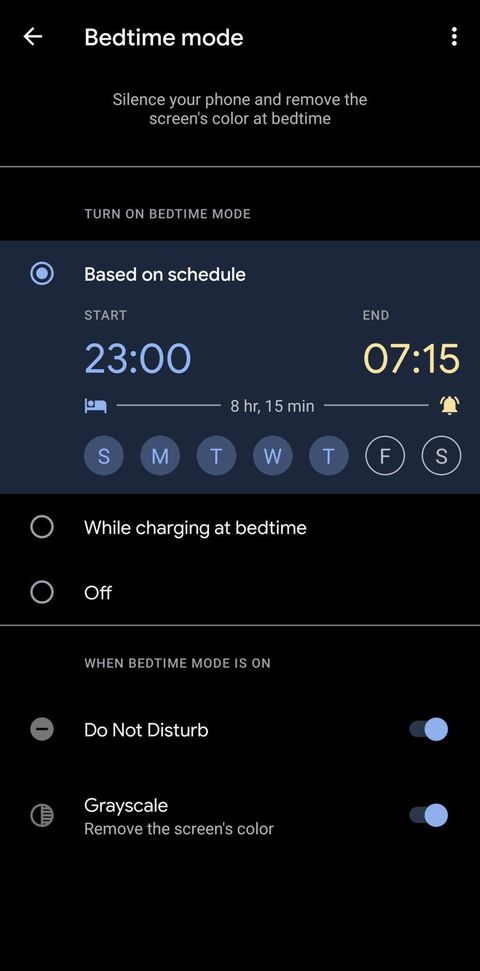**Detailed Caption:**

This screenshot displays a phone's Bedtime Mode settings, featuring a black background with white text for easy readability. Key details include:

- **Bedtime Mode Activation**: Enabled based on a custom schedule.
- **Schedule**: Starts at 23:00 (11:00 PM) and ends at 07:15 (7:15 AM), allowing for 8 hours and 15 minutes of designated sleep time.
- **Days Active**: The schedule applies daily from Sunday through Saturday.
- **Alarms**: All alarms are turned off.
- **Visual Indicators**: Start and end times are highlighted in light blue and light yellow, respectively.
- **Additional Settings**:  
  - The phone's screen displays black text on a white background while charging.
  - Bedtime Mode is currently off.
  - Do Not Disturb and Grayscale Mode (which removes color from the screen) are activated when Bedtime Mode is enabled, likely to discourage screen usage before sleep.
  
This feature is designed to promote better sleep habits by minimizing screen time and distractions at night.